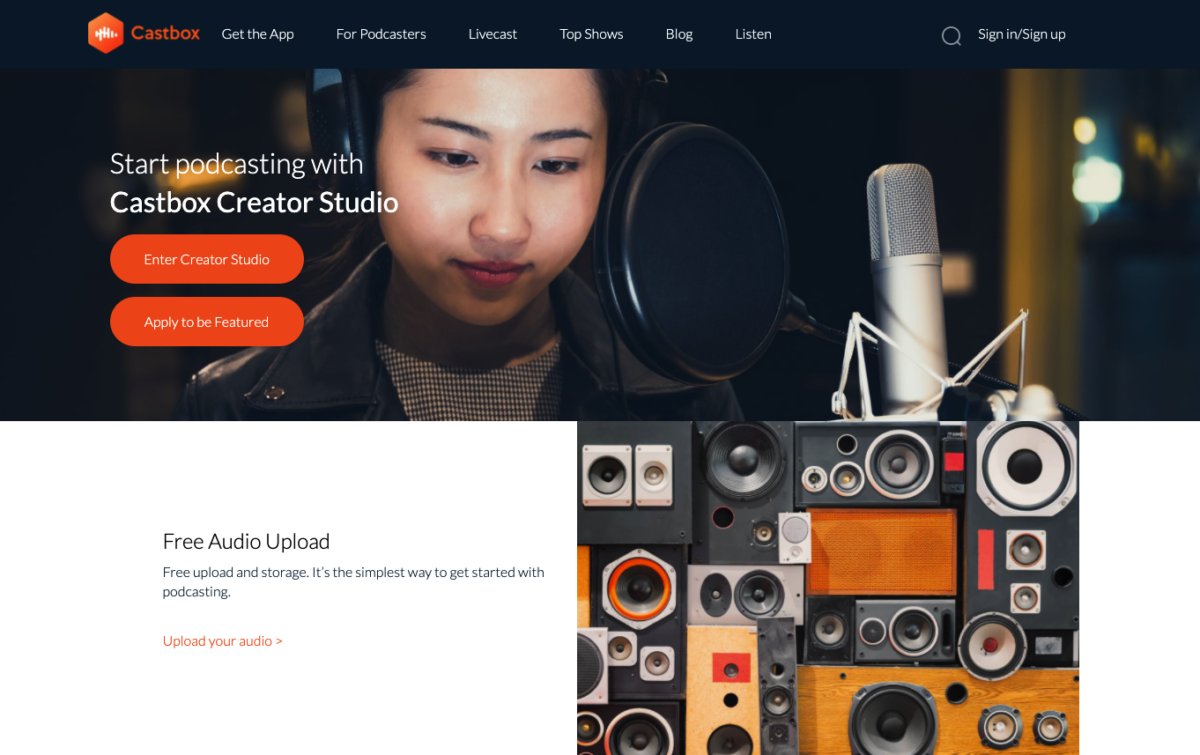Here's a detailed and clean caption:

"This screenshot captures the front page of CastBox, a podcasting platform. The CastBox logo, an orange hexagon with white sound wave bars, is prominently displayed in the top left corner. The navigation menu, which includes six tabs: 'Get the App,' 'Podcasters,' 'Livecasts,' 'Top Shows,' 'Blog,' and 'Listen,' is aligned horizontally across the top. In the top right corner, there are 'Sign In' and 'Sign Up' buttons. Below the header, an image features an Asian woman wearing headphones and speaking into a professional podcast microphone, with a pop filter placed between her and the mic. To the left of this image, white text reads, 'Start Podcasting with CastBox Creator Studios,' accompanied by two orange buttons labeled 'Enter Creator Studios' and 'Apply to be Featured.' Underneath this section, another image showcases an array of various computer and radio speakers stacked together. The accompanying text on the left side of this image states, 'Free Audio Upload, Free Upload and Storage,' followed by a red prompt, 'Upload Your Audio,' highlighting the platform’s user-friendly podcasting features."